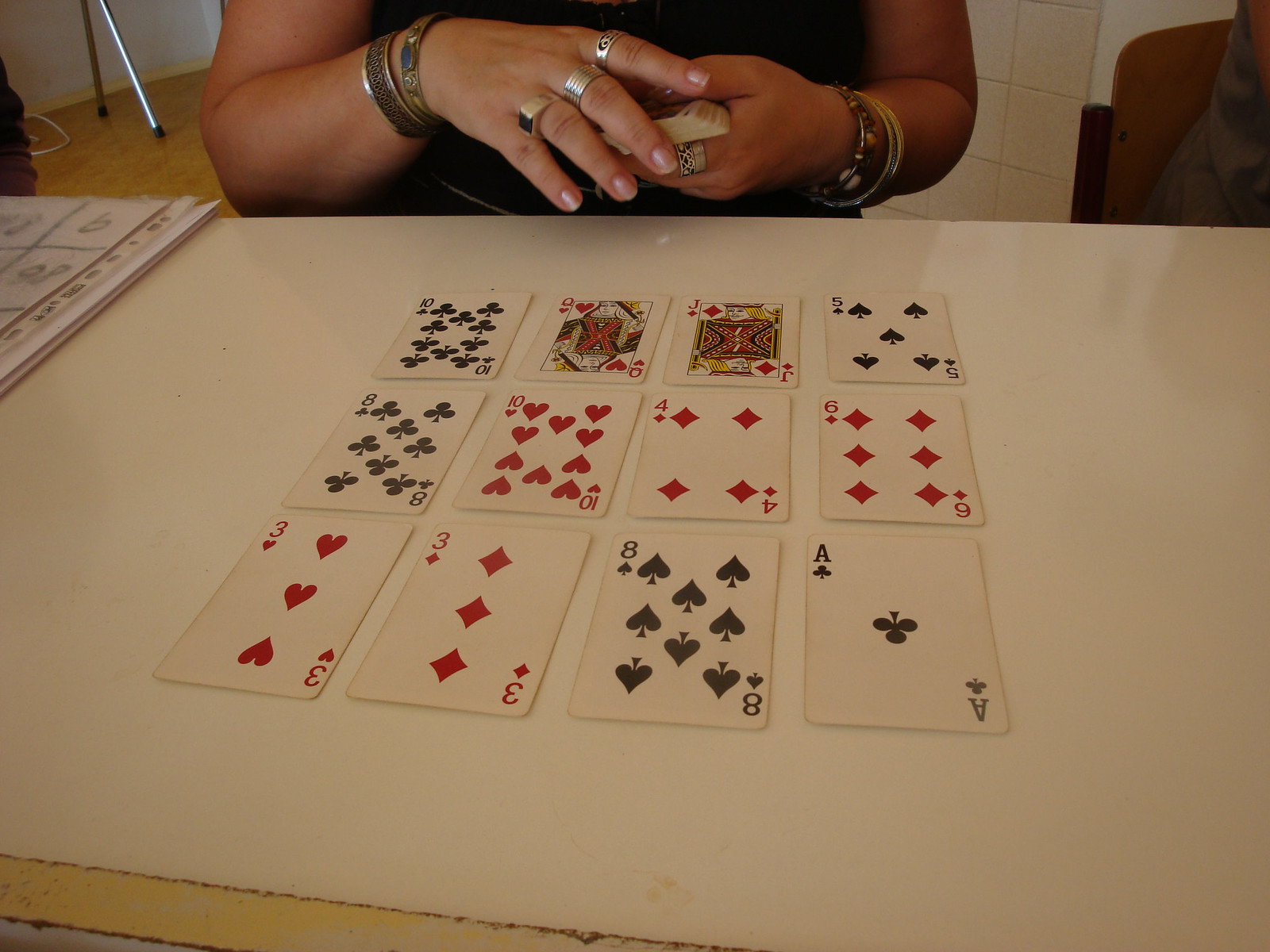In this detailed image, a woman is seated at a table, intently playing solitaire. She is positioned on an off-white chair, featuring a unique design with small square patterns. To her side, a brown chair is partially visible, draped in gray fabric that could either be a pillow or the clothing of a person seated there. The wall behind her is light-colored, and the legs of a small stand are apparent in the background. On her other side, another piece of cloth can be seen, suggesting the presence of another individual. The table is adorned with a white cloth, decorated with small printed squares that seem to display numbers.

The woman is dressed in a sleeveless dress and accessorized with multiple bracelets on each arm. On her left wrist, she wears a gold bracelet and another one that is a blend of gold and blue. Her left hand showcases three rings: two are silver, while the third is gold, featuring a large dark stone. On her right wrist, she dons three bracelets: two silver and one black, adorned with beads. She is captured in the act of shuffling cards, with twelve cards neatly laid out before her on the table.